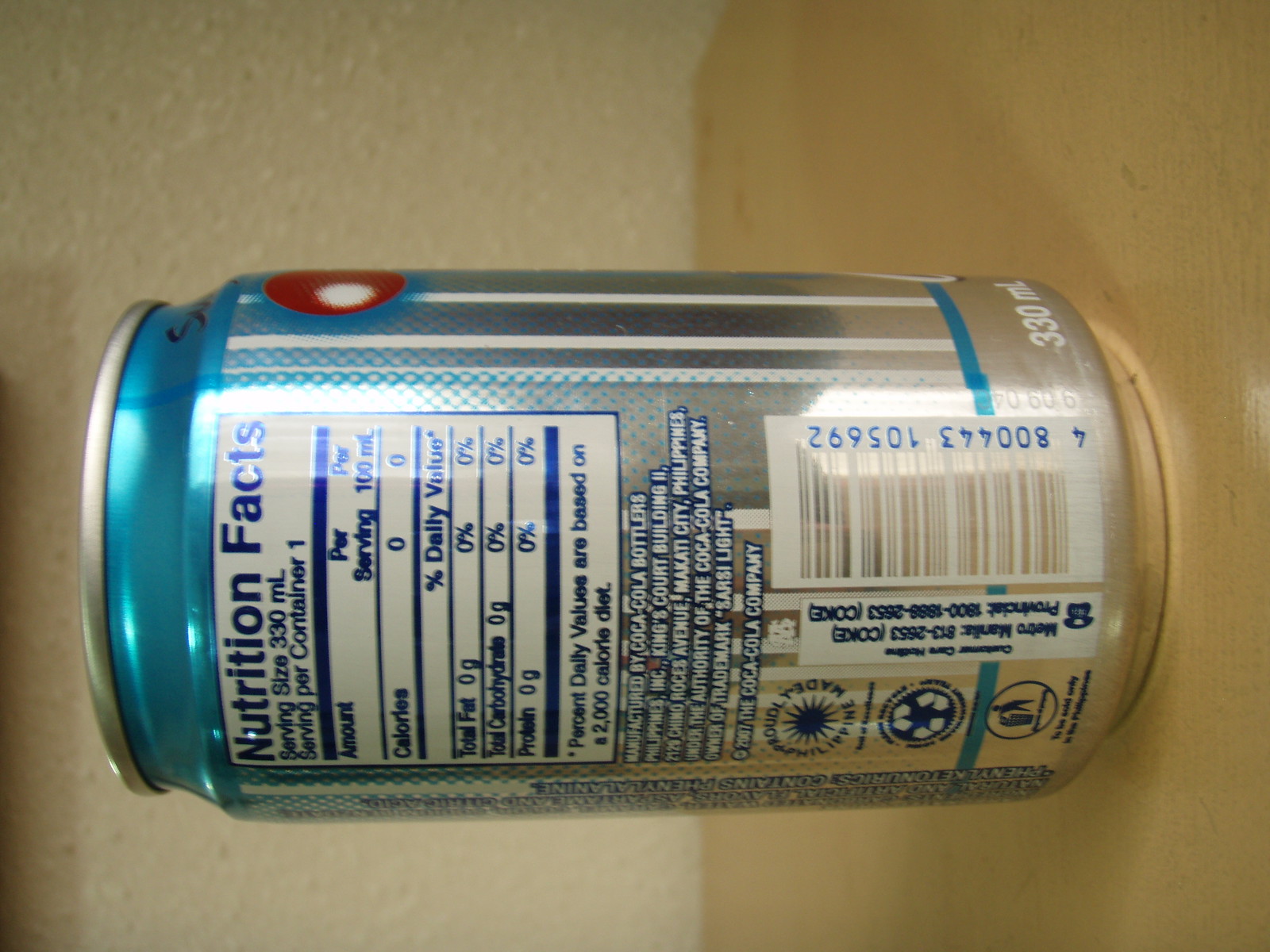The image depicts a can of a product that has been rotated to the left, making it appear as if the can itself is lying on its side. The top portion of the can features a shiny, silvery blue color that transitions downwards in a halftone effect, blending seamlessly with the silver base of the can. Prominently displayed is the can’s nutrition facts panel, which is designed with dark blue text on a white background, all encased within a solid blue border. The nutrition facts state: 

- Serving size: 330 milliliters
- Servings per container: 1
- Amount per serving: 100 milliliters
- Calories: 0
- Total Fat: 0 grams (0% DV)
- Total Carbohydrates: 0 grams (0% DV)
- Protein: 0 grams (0% DV)

It also includes a note that daily values are based on a 2,000-calorie diet. 

Below the nutrition facts are the ingredients list and manufacturing information, though the latter part is somewhat difficult to read due to the white text with blue outline. The can is manufactured by Coca-Cola Bottlers. Adjacent to this information is a barcode and several recycling symbols. The can is placed on a light brown wooden surface, with a neutral wall serving as the backdrop. There are no other objects or elements in the image, ensuring full focus remains on the can.